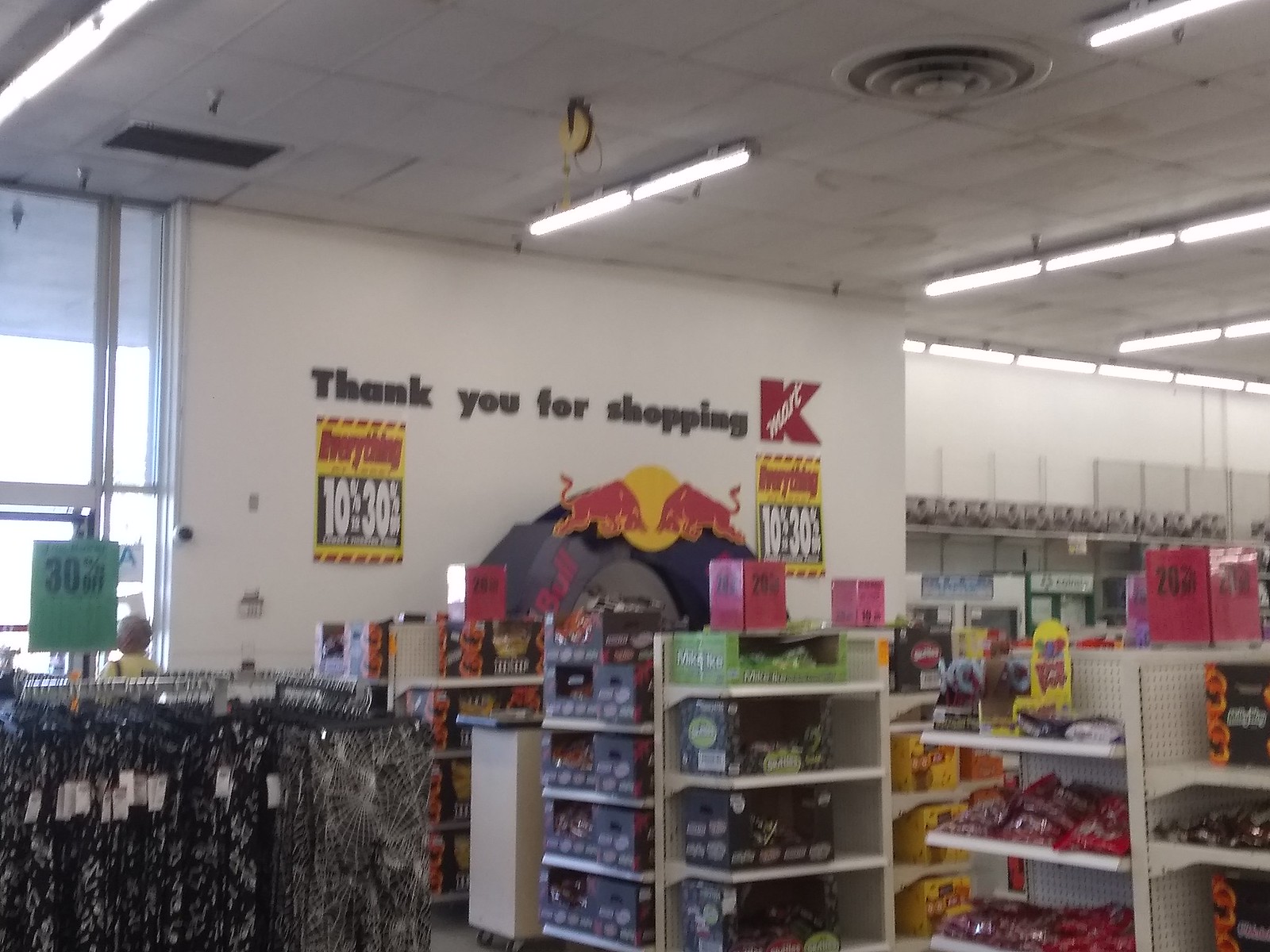This image, though blurry, captures an interior scene of a Kmart store. The focal point is a white wall prominently displaying the store's iconic branding: a large red "K" with the word "Mart" in white letters within the "K." Directly above this logo, black letters spell out "Thank you for shopping Kmart." Below this permanent signage, there are temporary yellow signs with red writing, accompanied by black banners indicating a sale ranging from 10% to 30% off. The text on the banner reads "Everything" in bold red letters against the bright yellow background. To the right of the image, steel shelves are visible, adorned with a variety of snack foods. On the left, hanging pants are displayed on a rack beneath a green sign that also advertises 30% off in black letters. In the background, we can discern the tall glass entranceway of the store.